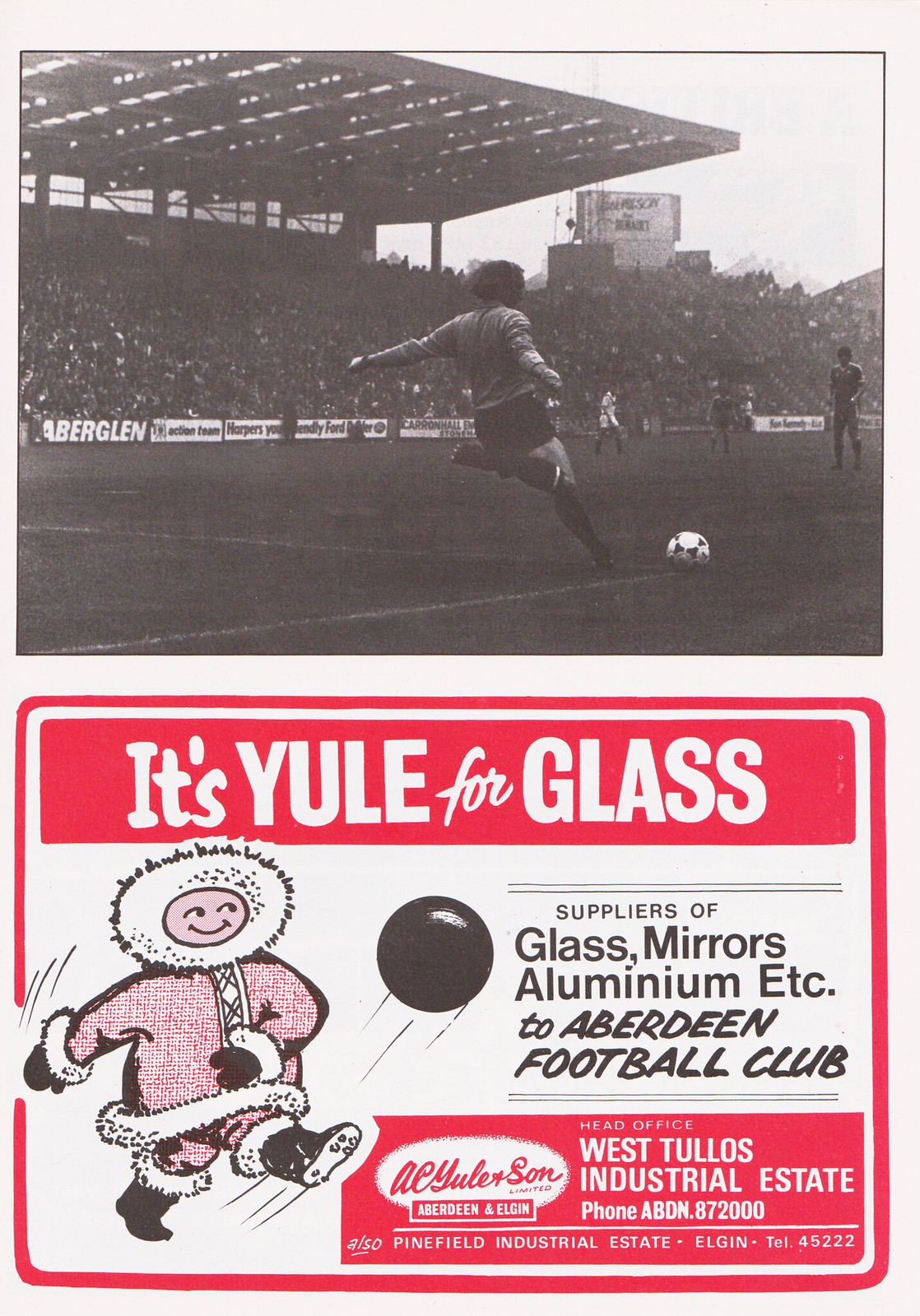This vintage advertisement features a nostalgic black and white photo at the top, showcasing a dynamic soccer match. The image captures a soccer player in black shorts and socks, poised to kick a black and white ball, with a sizable audience of approximately 300-400 spectators in the stands. The crowd sits under a covered area, adding to the lively atmosphere. In the background, there are white signs on a wall behind the spectators, including partially visible text such as "Aberglen" and "Wilson."

Below the photograph, a vibrant red and white advertisement prominently displays the text "It's Yule for Glass." The central illustration in the ad depicts a figure in an Eskimo outfit, complete with a fur-trimmed hood, long coat, pants, and boots, all in red with black and white detailing. The Eskimo appears to be kicking a black ball, reinforcing the soccer theme.

The advertisement further highlights that the company is a supplier of glass, mirrors, aluminum, etc., to Aberdeen Football Club. Additional text provides contact information for the company's offices: the head office at West Toulouse Industrial Estate (Phone ABDN 87200) and another location at Penfield Industrial Estate, Elgin (Phone 45222). The company name, A.C. Euler & Son, is prominently displayed, indicating their involvement in supporting the football club.